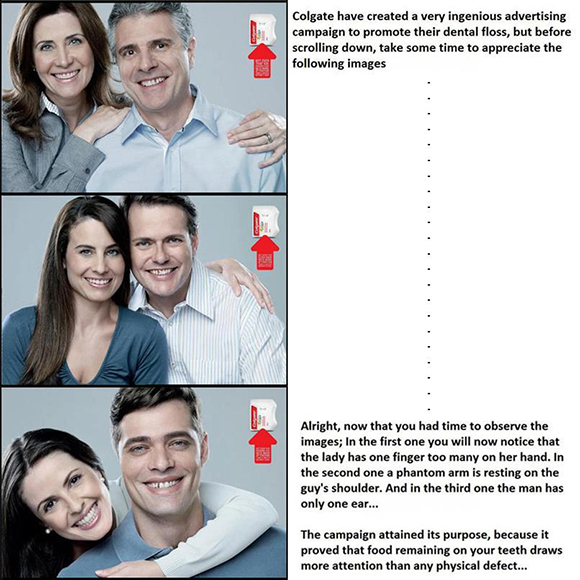This image is part of a clever Colgate advertisement campaign designed to promote their dental floss. It features three photos arranged in a vertical grid, each depicting a man and a woman. At first glance, the most noticeable detail is that the man in each photo has a piece of food stuck in his teeth. However, upon closer inspection, several unusual physical defects are evident in the images: in the top photo, the woman has an extra finger on her right hand; in the middle photo, a phantom arm inexplicably appears around the man’s shoulder; and in the bottom photo, the man is missing his right ear. The text to the right of the images reads, "Colgate has created an ingenious advertising campaign to promote their dental floss. Before scrolling down, take some time to appreciate the following images. Now that you’ve had time to observe, you will notice the lady has one finger too many, a phantom arm is resting on the guy's shoulder, and the man has only one ear. The campaign achieves its purpose by proving that food stuck in your teeth draws more attention than any physical defect." The ad's background colors are predominantly white, black, red, and blue, suggesting it may be a social media post.